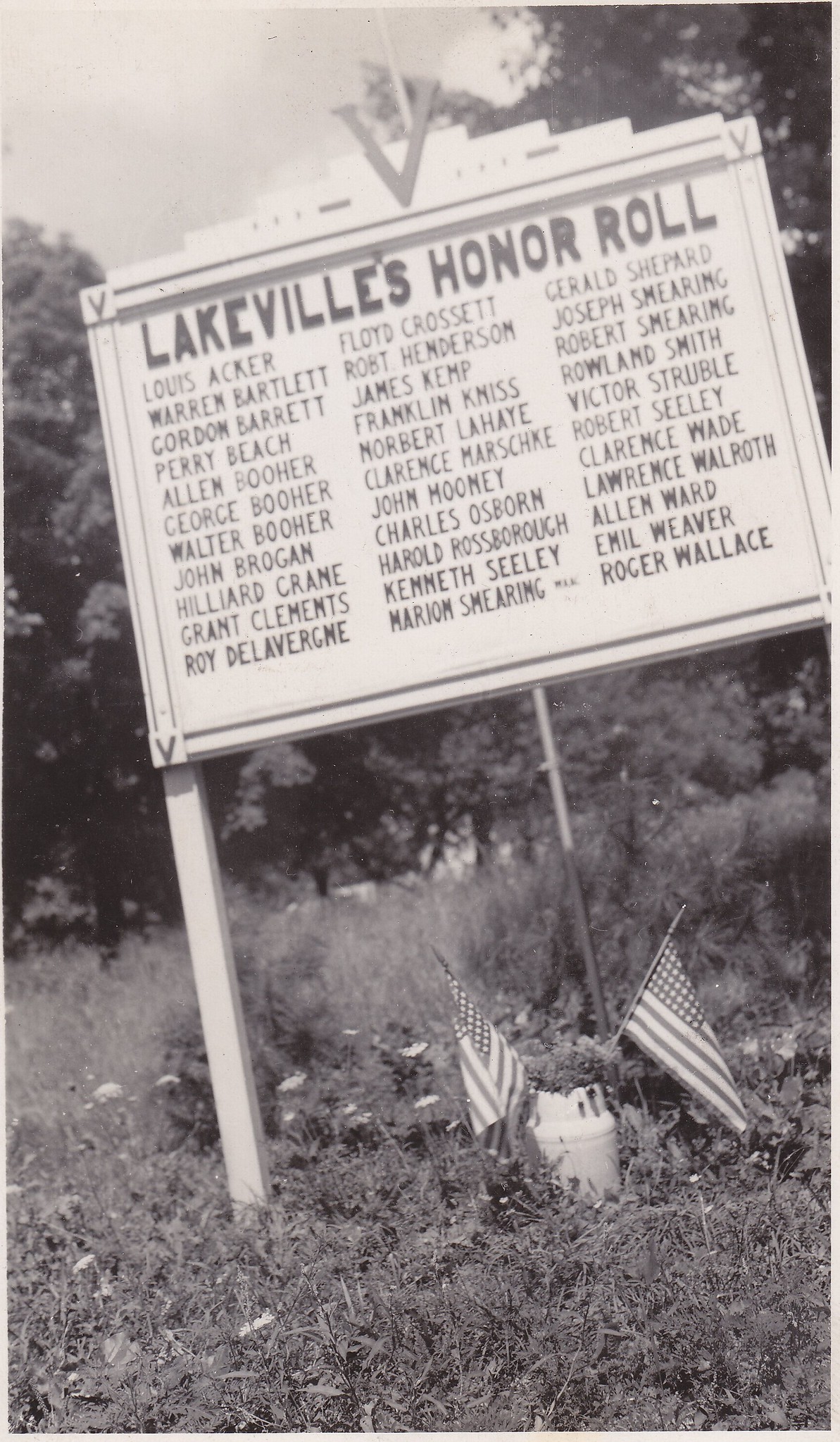This black and white photograph captures an old monument situated outdoors, surrounded by vegetation. The central feature is a large wooden sign with dark lettering set against a white background, mounted on posts. Dominating the top of the sign is a large "V," followed by the bold heading "Lakeville's Honor Roll." The sign lists three columns of names, although they are somewhat hard to read. The names include Lewis Acker, Warren Bartlett, Gordon Bartlett, Perry Beach, Alan Bucher, George Bucher, Walter Bucher, John Brogan, Hilliard Crane, Grant Clements, Roy Delaverne, Flores Floyd Gap Crosset, Robert Henderson, James Kemp, Franklin Niss, Norbert Lahey, Clarence Marshke, John Mooney, Charles Osborne, Harold Rossoborough, Kenneth Seeley, Marion Smearing, and Roger Wallace.

Beneath the sign, there is a small pot with two American flags protruding from it, and the area around the sign is somewhat overgrown with weeds and wildflowers. The background reveals a tree or trees, and the sky, visible in the upper left-hand corner of the image, is gray and cloudy.